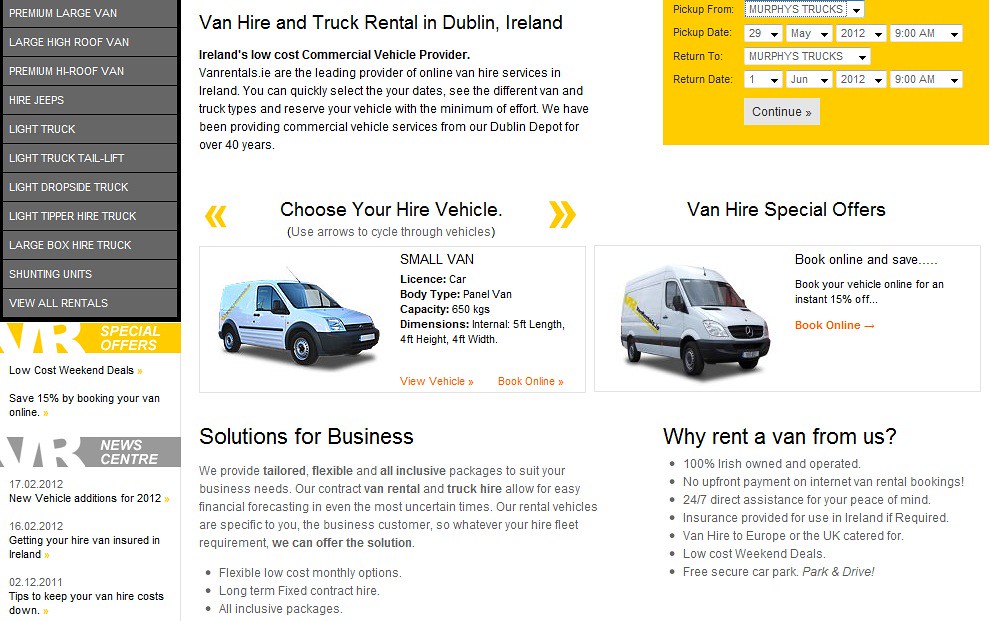This screenshot captures the homepage of a van hire and truck rental service based in Dublin, Ireland. On the left-hand side, a gray rectangular box lists various vehicle options, including Premium Large Van, Large High Roof Van, Premium High Roof Van, Hire Jeeps, Light Truck, Light Truck with Tail Lift, Light Drop Side Truck, Light Tipper Hire Truck, Large Box Hire Truck, Shunting Units, and a link to view all rentals.

Beneath this list, a prominent yellow bar highlights special offers, including low-cost weekend deals and a promotion to save 15% by booking online. Directly below, a gray rectangle features announcements about the company's new center, new vehicles, additions for 2012, advice on getting hire van insurance in Ireland, and tips for reducing van hire costs.

The central section of the page proudly states, "Ireland's Low Cost Commercial Vehicle Provider." It further explains that VanRentals.ie is a leading provider of online van hire services in Ireland, allowing users to easily select dates, browse various van and truck types, and reserve vehicles with minimal effort. The company boasts over 40 years of experience in supplying commercial vehicles and services from their Dublin depot.

In the top right corner, a yellow box presents options for scheduling, including fields for 'Pickup From,' 'Pickup Date,' 'Return To,' and 'Return Date,' helping users plan their rentals efficiently.